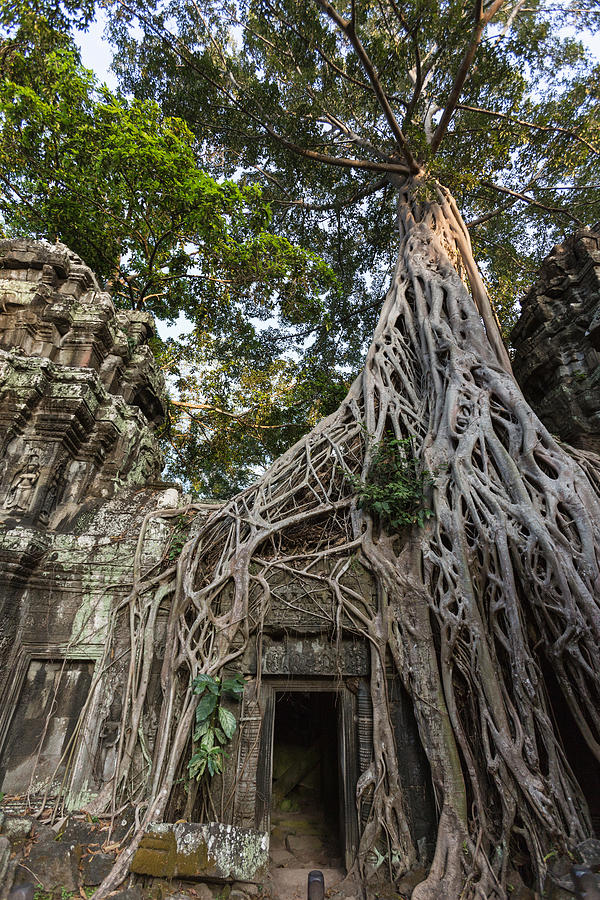The image depicts an ancient, decrepit stone temple that has been overtaken by nature, predominantly by the root system of a towering tree located on the right-hand side. The roots, which are a light brown color, cascade down from the upper part of the temple, draping over the structure like flowing liquid and intertwining with the white stones. The temple, set within a dense forest, features an entrance prominently at the bottom center of the image, leading into darkness, making it unclear what lies inside. The building is intricately etched with detailed patterns, figures of women, and elaborate designs around doorways, showcasing lichen deposits and a grungy appearance indicative of long-term abandonment. Through the trees above, a bit of sky is visible, suggesting that the photo was taken during daylight, possibly in the late afternoon.